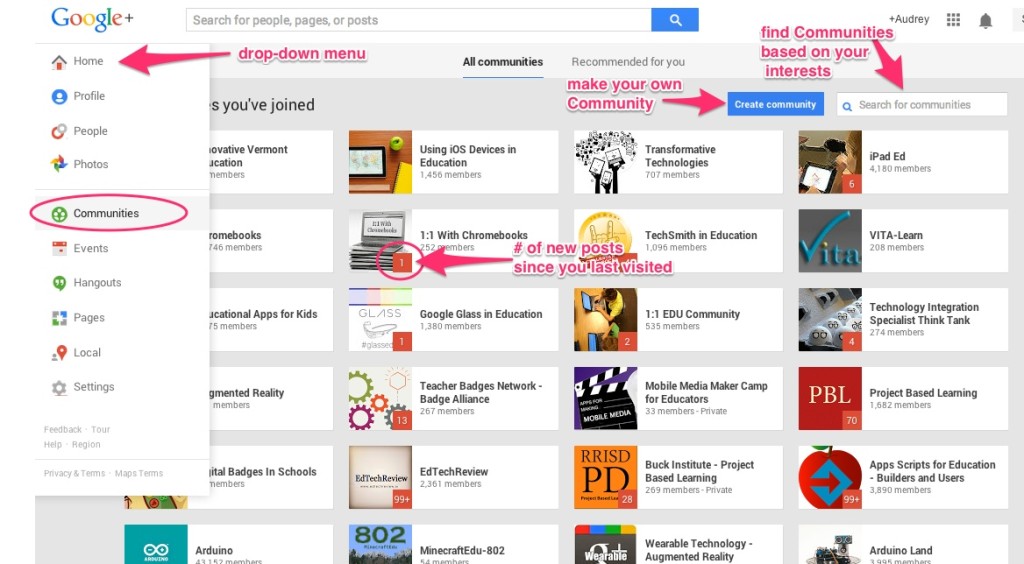Screenshot Tutorial for Navigating Google+ Communities Interface:

The image is a screenshot of the Google+ interface, focusing on the Google account's community management features. This screenshot is used as a tutorial, annotated with hot pink arrows and text for clarity. The background of the interface is pale grey with multiple white rectangles, each containing a thumbnail on the left and descriptive text on the right. 

On the left side, under the word "Google+", there's a visible drop-down menu that includes options like Home, Profile, People, Photos, Communities, Events, Hangouts, Pages, Local (with a map symbol), and Settings. The search bar at the top is empty.

Key annotations and elements of the tutorial include:

1. **Home Menu**: The first hot pink arrow points to the word "Home" in the drop-down menu, with the key text "Drop-down menu" for clarification.

2. **Create Community Button**: At the top right of the image, there is a prominent blue button labeled "Create Community". Next to this button, there's an empty text box labeled "Search for communities". An arrow directs the viewer's attention to the text box with the key "Find communities based on your interests." Another arrow points to the "Create Community" button with the key "Make your own community."

3. **Highlighted Communities Option**: In the left drop-down menu, the word "Communities" is circled in hot pink, emphasizing its importance in the tutorial.

4. **New Post Notification**: In the second column from the left on the second row down, there's a community highlighted with a notification number. A hot pink arrow points from right to left, directing attention to the circled notification, with the key "Number of new posts since you've last visited."

5. **Community Grid**: The rest of the interface displays a grid consisting of four columns and six rows of community thumbnails and descriptions, representing the communities followed by the user through their Google account.

This detailed caption provides a comprehensive guide to understanding the various elements and annotations included in the tutorial screenshot.